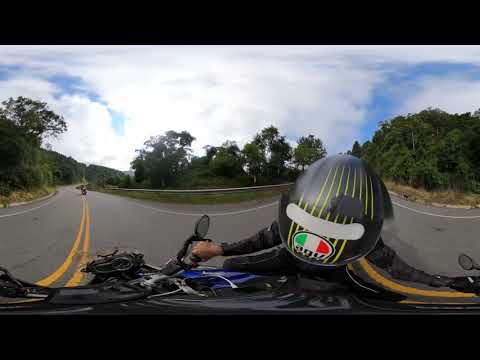An immersive image captures the dynamic moment from the vantage point of a vehicle’s dash cam, featuring a scene that could either be a snapshot of a potential accident or an unusual perspective of a motorcycle ride. The image portrays a two-lane road on the left, divided by a double yellow line, bordered by trees on both sides. Due to a distorted lens, the road appears curved and twisted, adding an almost surreal effect to the scene. In the foreground, the top section of a motorcyclist is prominently visible, including the helmet, right arm, hand, and the upper part of the motorcycle. The motorcyclist, who appears to be female based on body language and hand posture, might be capturing the scene with a selfie camera, creating an odd juxtaposition as they ride on this open country road. The upper third of the photograph is dominated by clouds with a few patches of blue peeking through, completing the atmospheric setting of this intriguing and somewhat ambiguous moment on the road.